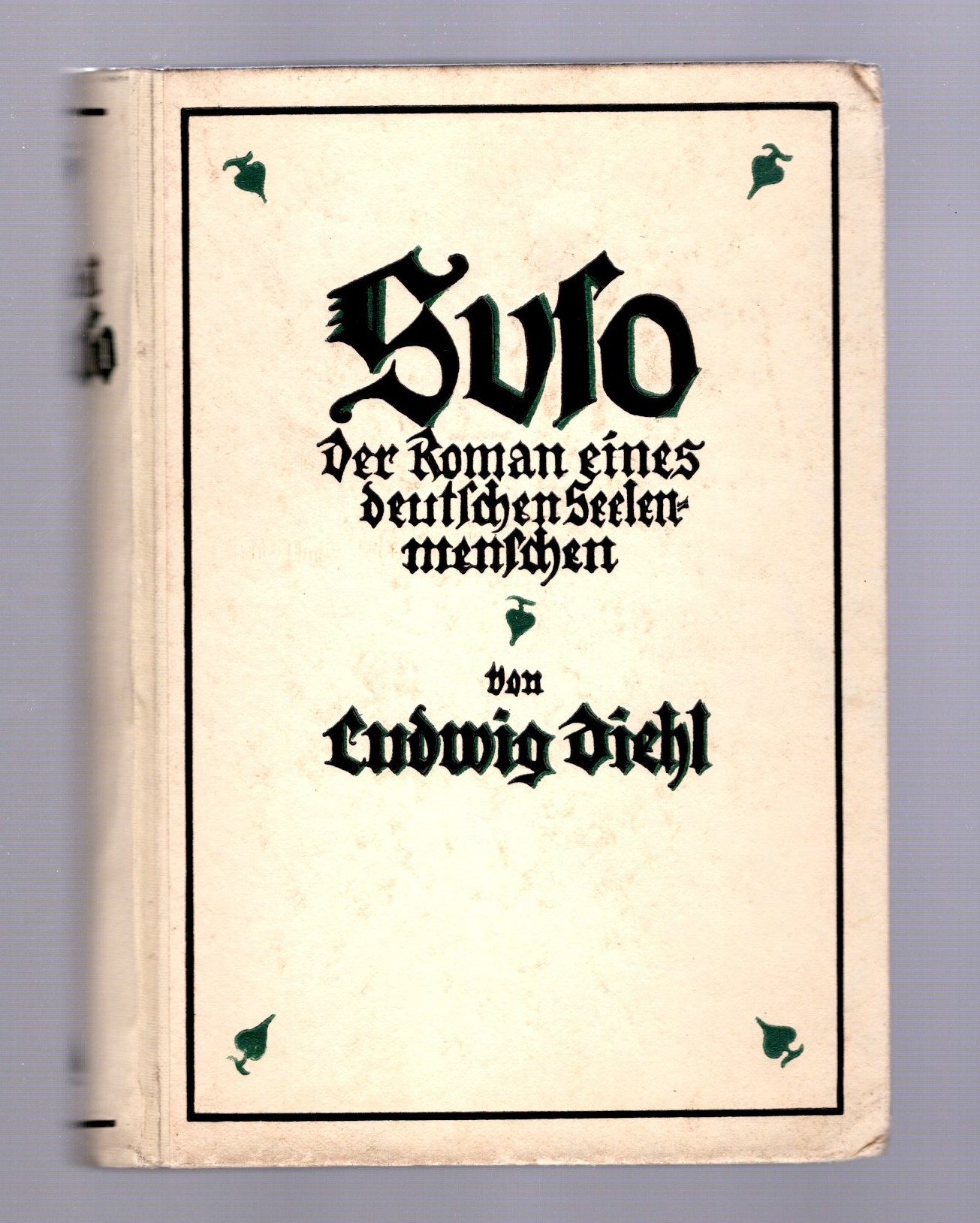The image features an old German book placed on a flatbed scanner with a lilac background. The book has a white, slightly aged, leather cover with a thin black rectangular border framing the front. Ornate details include four small ace symbols, resembling those from a deck of cards, positioned near each corner and pointing towards the center of the cover. The title, written in a style that mimics old German script and appears almost handwritten, reads "SUSO. Der Roman eines deutschen Seelenmenschen," which translates to "Suso: The Novel of a German Human Soul." The author is Ludwig Diehl. The book shows signs of wear, with bent corners and slight darkening, suggesting its age and usage.